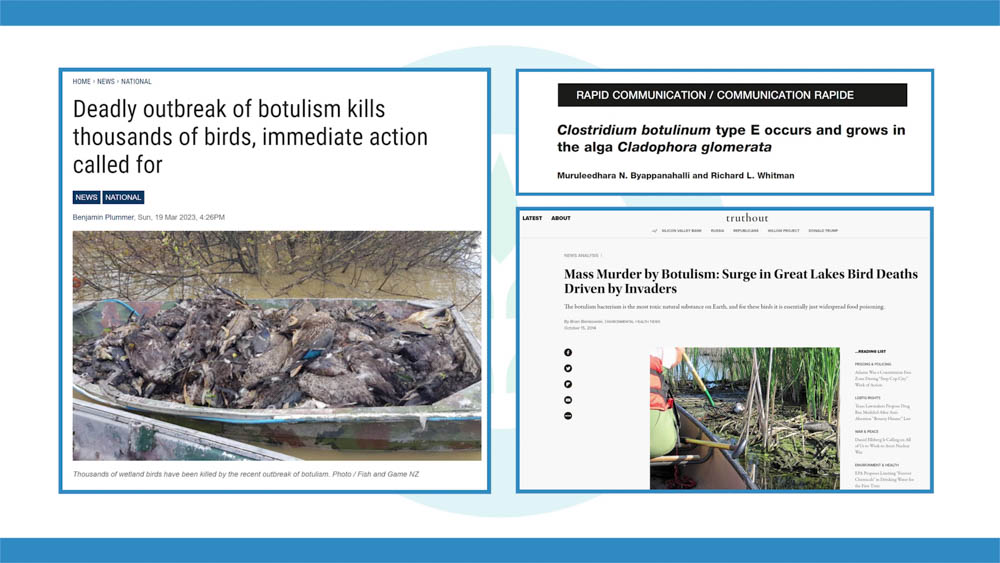**Descriptive Caption:**

This image is a screenshot of a news webpage featuring multiple articles about a severe botulism outbreak affecting bird populations. The top of the page is marked by a blue border stretching across its entirety, devoid of any text. The left side is dominated by a main article enclosed in a blue border, titled "Home News National." The article's headline reads: "Deadly Outbreak of Botulism Kills Thousands of Birds. Immediate Action Called For."

Beneath this headline, there is an unsettling image showing a heap of dead birds piled in what appears to be a boat, situated outdoors. The photo's caption reads: "Thousands of Wetland Birds Have Been Killed by the Recent Outbreak of Botulism."

To the right of the main article, there are two rectangular sections with blue borders housing brief news snippets. The first rectangle, labeled "Rapid Communication / Communication Rapide" in both English and French, provides a brief scientific note: "Clostridium botulinum, type E, occurs and grows in the alga Cladophora glomerata."

Below this, another rectangle is labeled "Truth Out" at the center of its top. This section previews an article with the headline: "Mass Murder by Botulism, Surge in Great Lakes Bird Deaths Driven by Invaders." The associated photo shows a blurry depiction of wetlands with a person partially visible in a boat; the image is unclear but appears to include bird bodies.